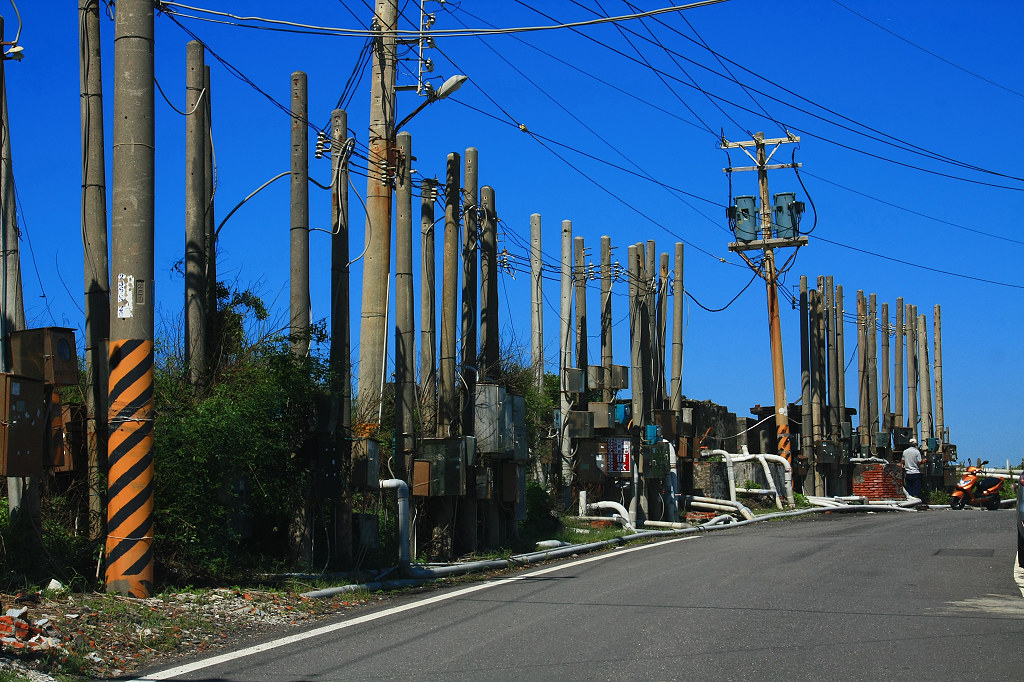The image is a color photograph taken outdoors, featuring a strikingly vibrant, digitally enhanced blue sky that spans the upper half of the frame. Below this sky, a row of tall, large poles with wide circumferences line a concrete or asphalt road, stretching diagonally from the top left to the bottom right corner. The poles, primarily black and metallic in appearance, support a tangled web of black wires crisscrossing the sky. One of the poles is distinctive, wrapped with a sticker displaying orange and black diagonal spirals.

At the far end of the road sits an orange motorcycle or moped, parked almost touching the right edge. Nearby, the back of a person in a white short-sleeve t-shirt, dark pants, and possibly a white hat or hardhat can be spotted. The scene also includes some greenery, with patches of grass and pebbles, and scattered debris, suggesting a somewhat cluttered environment. A semblance of construction activity, indicated by distant workers and some construction equipment, enhances the complexity of the scene.